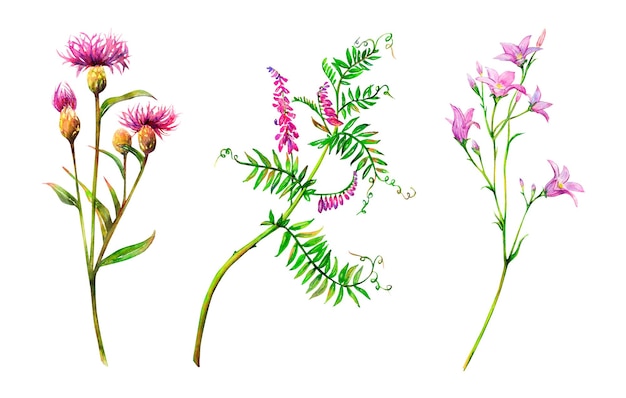The illustration showcases three elegantly depicted botanical specimens against a pristine white background, resembling detailed botanical drawings that have been expertly sketched and painted. Each plant features stems, leaves, and vibrant flowers, rendered with such realism they almost leap off the page.

On the left, a thistle-like plant with dark green, narrow oval leaves branches into a V-shape. Its stems culminate in dense clusters of dark yellow, bulbous flower bases crowned with spiky, feather-like hot pinkish-purple petals that radiate outward in a wild, eye-catching display.

The central plant seems characteristic of a wild pea, with a long, arching green stem adorned with numerous fern-like leaves. Slender and delicate, its funnel-shaped pea flowers branch off on thin stems, each bloom composed of many tiny purple petals that line the length of the stem.

To the right, the final plant resembles a lily with thin, curving stems that bear tiny, nearly invisible leaves. At the ends of its branches, trumpet-shaped flowers with creamy white and soft purple hues stand out, each bloom bearing six petals that fan out gracefully, resembling a bell as they open broadly into flat edges.

Together, these three plants form a captivating and detailed botanical study, presenting a harmonious blend of color and form.